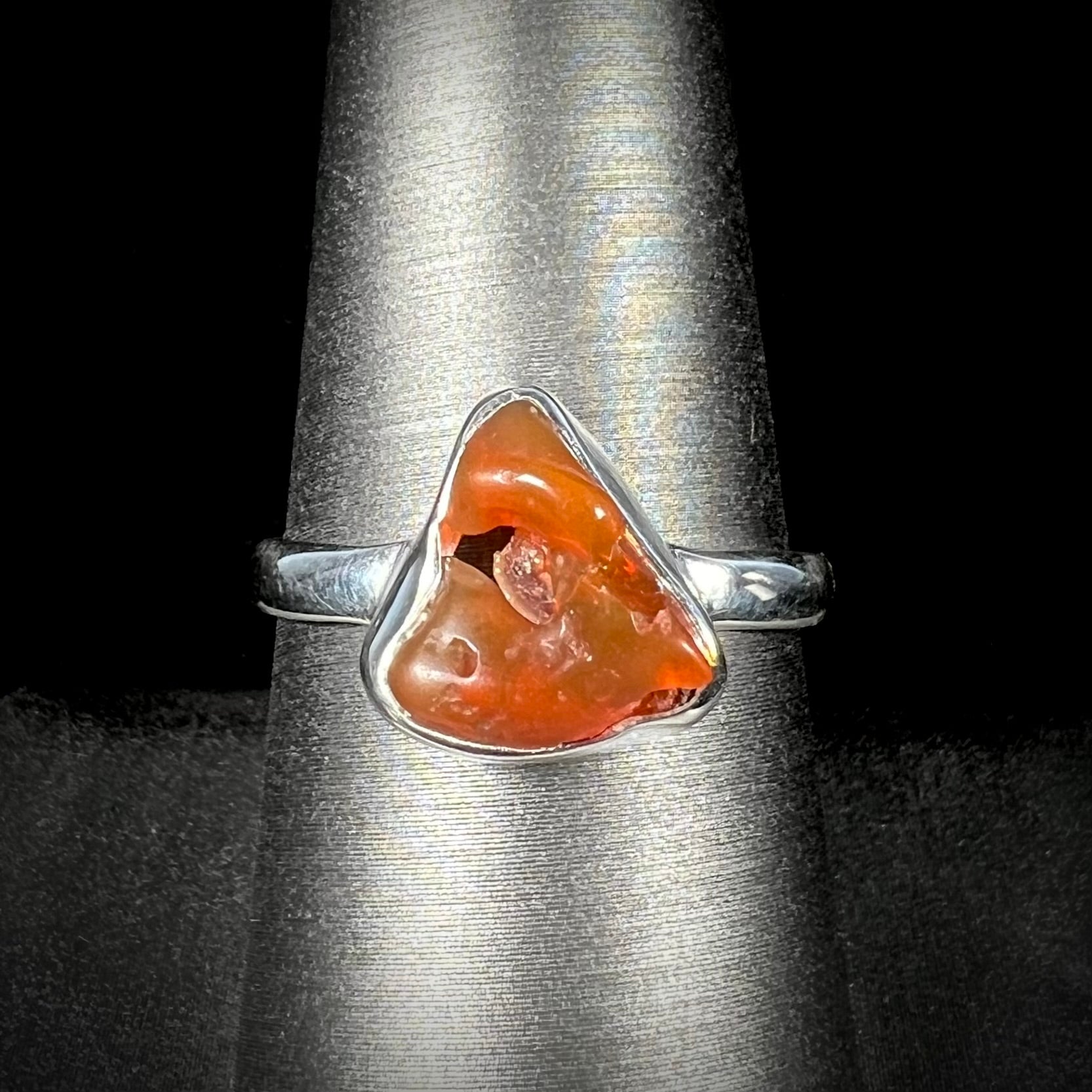This detailed color photograph captures a silver ring placed on a metallic, conical object that resembles a ring sizer or perhaps a soldering iron. The bright, shiny silver ring, which appears handcrafted, features a central orange triangular gemstone that has the appearance of melting gelatin. The gemstone, likely carnelian or agate, reveals a glossy, slightly irregular surface that forms a contrast against the smooth metal band. The conical object behind the ring, which could be some kind of heat source, displays a tiny helical screw pattern, visible upon close zoom. The background of the image is predominantly dark, with the top half solid black and the bottom half a dark gray shade, enhancing the focus on the ring and its intriguing composition.